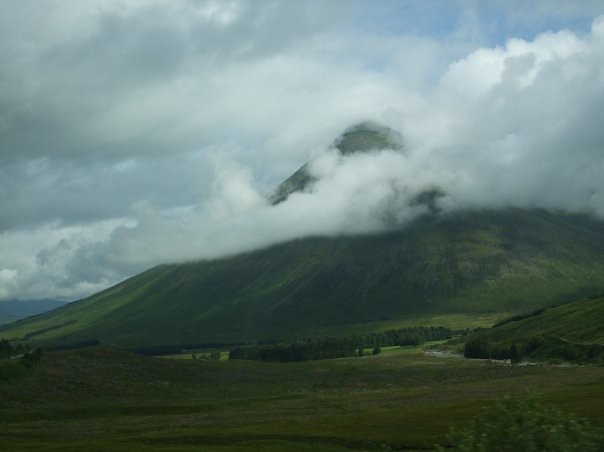The image is a detailed depiction of a vast, lush countryside dominated by a solitary, conical hill covered in dense forest. This isolated mount, standing alone with an estimated height between 2,000 and 3,000 feet, pierces through a sea of white, puffy clouds or low-lying fog, which envelopes the landscape, adding to its ethereal beauty. Below the hill, the valley sprawls out in vibrant green, nourished by the moisture-rich clouds that hover above. Nestled within this green expanse is a small, shallow lake, enhancing the serene, natural beauty of the vista. In the upper background, dark, rain-laden clouds add a dramatic contrast to the otherwise tranquil scene, hinting at an impending storm. Although resembling a photograph, the meticulous detail gives it a painterly quality, with the clouds seemingly in motion from left to right. This countryside panorama, absent of any artist’s signature, captures the striking, verdant beauty and solitude of this unique landscape.